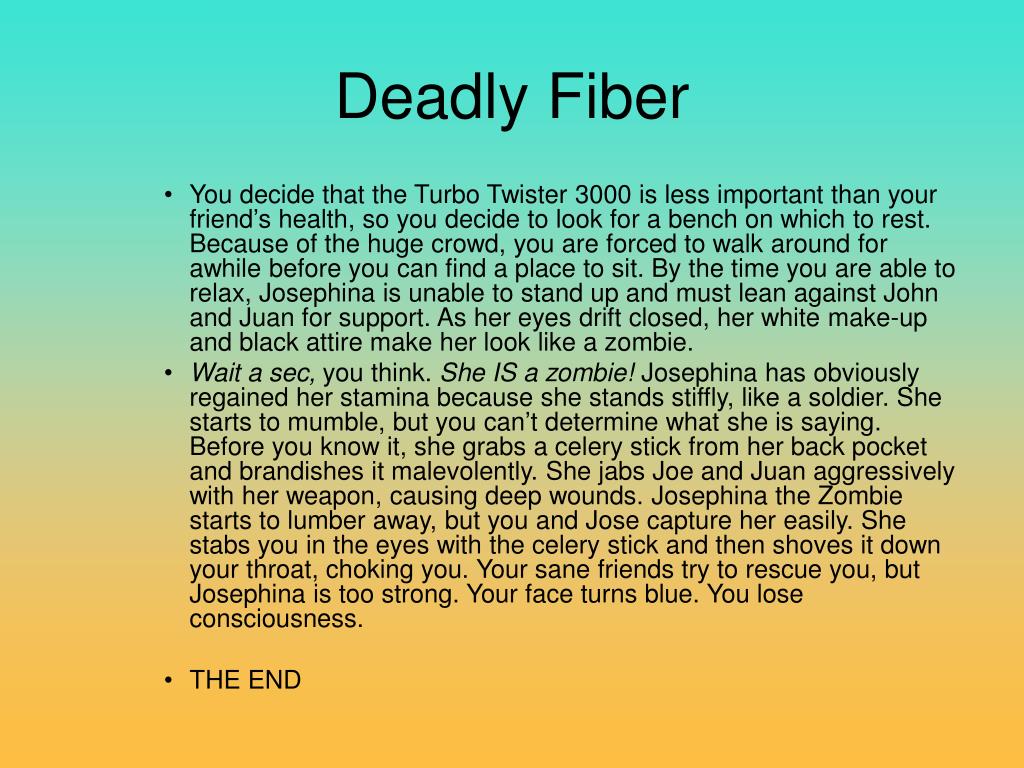The image is a PowerPoint slide featuring a gradient background that transitions from bright teal at the top to goldenrod at the bottom. The title "Deadly Fiber" is prominently displayed at the top in large, black sans-serif font. The slide contains three bullet points. The first bullet point narrates that you prioritize your friend's health over the Turbo Twister 3000 and decide to look for a bench to rest. Due to the crowded environment, it takes a while to find a place to sit. By the time you can relax, Josefina can no longer stand and must lean on John and Juan for support. Her white makeup and black attire make her appear zombie-like as her eyes drift closed. The second bullet point reveals that Josefina is indeed a zombie; she regains her stamina, stands stiffly like a soldier, and begins to mumble incoherently. Suddenly, she retrieves a celery stick from her back pocket and brandishes it aggressively, inflicting deep wounds on John and Juan. Although she begins to lumber away, you and Jose manage to capture her, but she viciously stabs you in the eyes with the celery stick and then shoves it down your throat, choking you. Despite your friends' attempts to rescue you, Josefina's strength overwhelms them. Your face turns blue, and you lose consciousness. The final bullet point concludes with "THE END" in all caps.